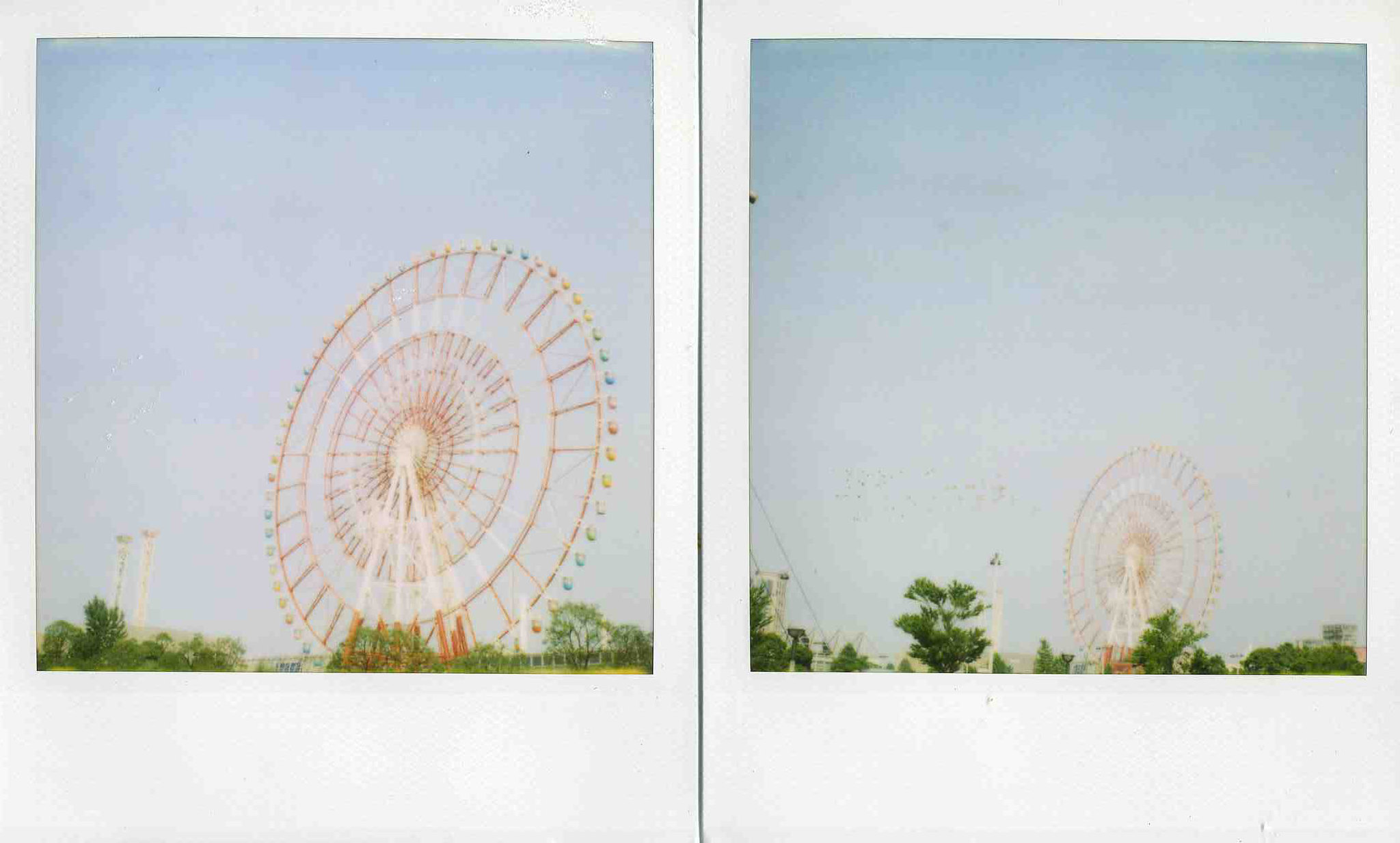This image showcases two Polaroid pictures placed side by side, each featuring the same Ferris wheel against a clear blue sky. Both photographs are framed with the classic white Polaroid border. The primary distinction between the two is that the one on the left is a close-up, providing a detailed view of the Ferris wheel's intricate elements, individual seats, and the red spokes within a white tripod-like structure. In contrast, the right photo is taken from a further distance, offering a broader perspective that includes power lines and a tree line dotted with various green trees and plants at the bottom. The Ferris wheel, prominent in both shots, has an orange framework with seats in multiple colors, and a tower structure can be seen off to the left of the Ferris wheel in both images.